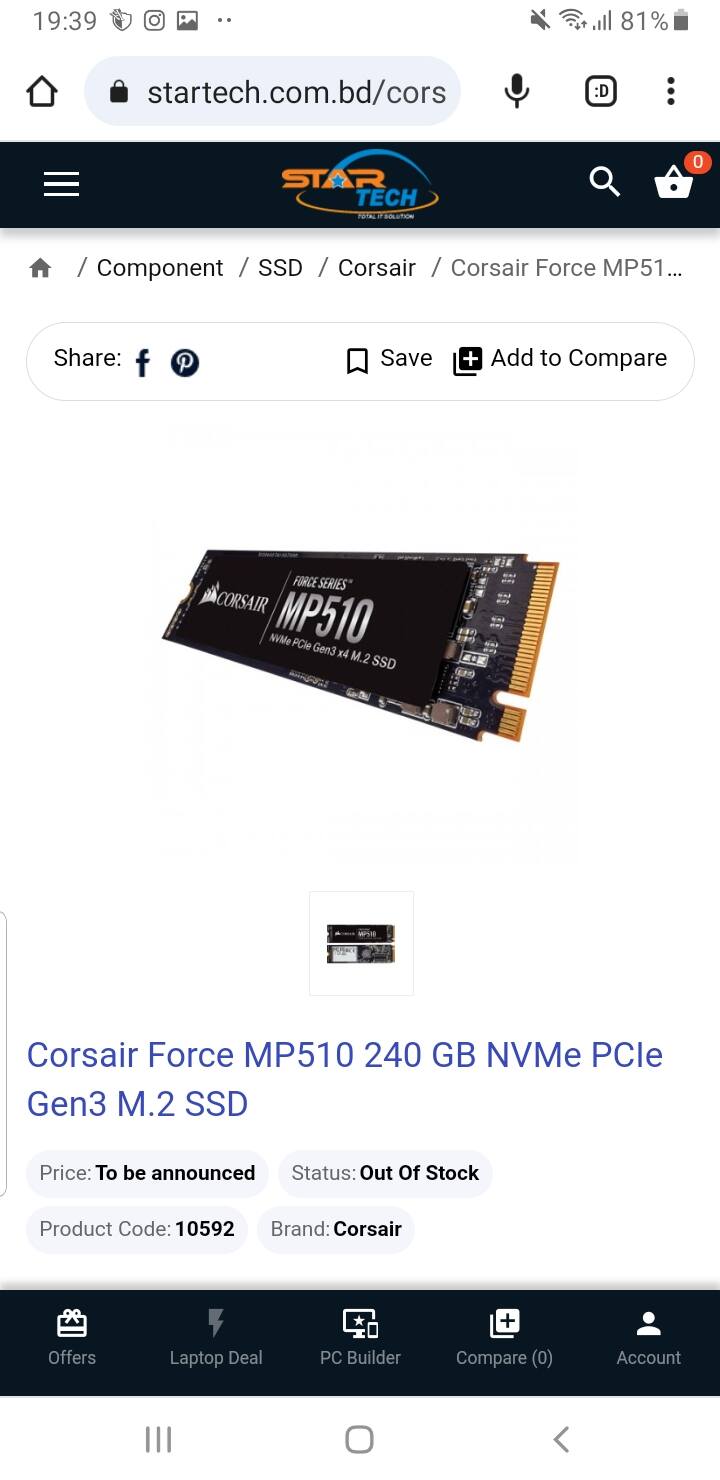Displayed on a mobile phone screen is the StarTech.com website. At the very top, the phone interface shows the time, along with icons for photos, the camera, sound off, Wi-Fi, phone service, and an 81% battery charge indicator.

Beneath this interface, the URL address bar contains "StarTech.com.pd/cors" with an array of icons, including a microphone, tab management, and a menu represented by three dots. 

The website itself has a dark blue color scheme with the "Star" part of the brand name in orange font, and "Tech" in blue font. The page features an image of the Corsair Force MP510 240GB NVMe PCIe Gen 3 SSD card. Below the image, details are provided: "Price: To be announced," "Status: Out of stock," "Product Code: 10592," and "Brand: Corsair."

Towards the bottom of the page, a navigation bar displays offers for "Laptop Deals," "PC Builder," "Compare," and "Account," all in white text set against a dark blue background.